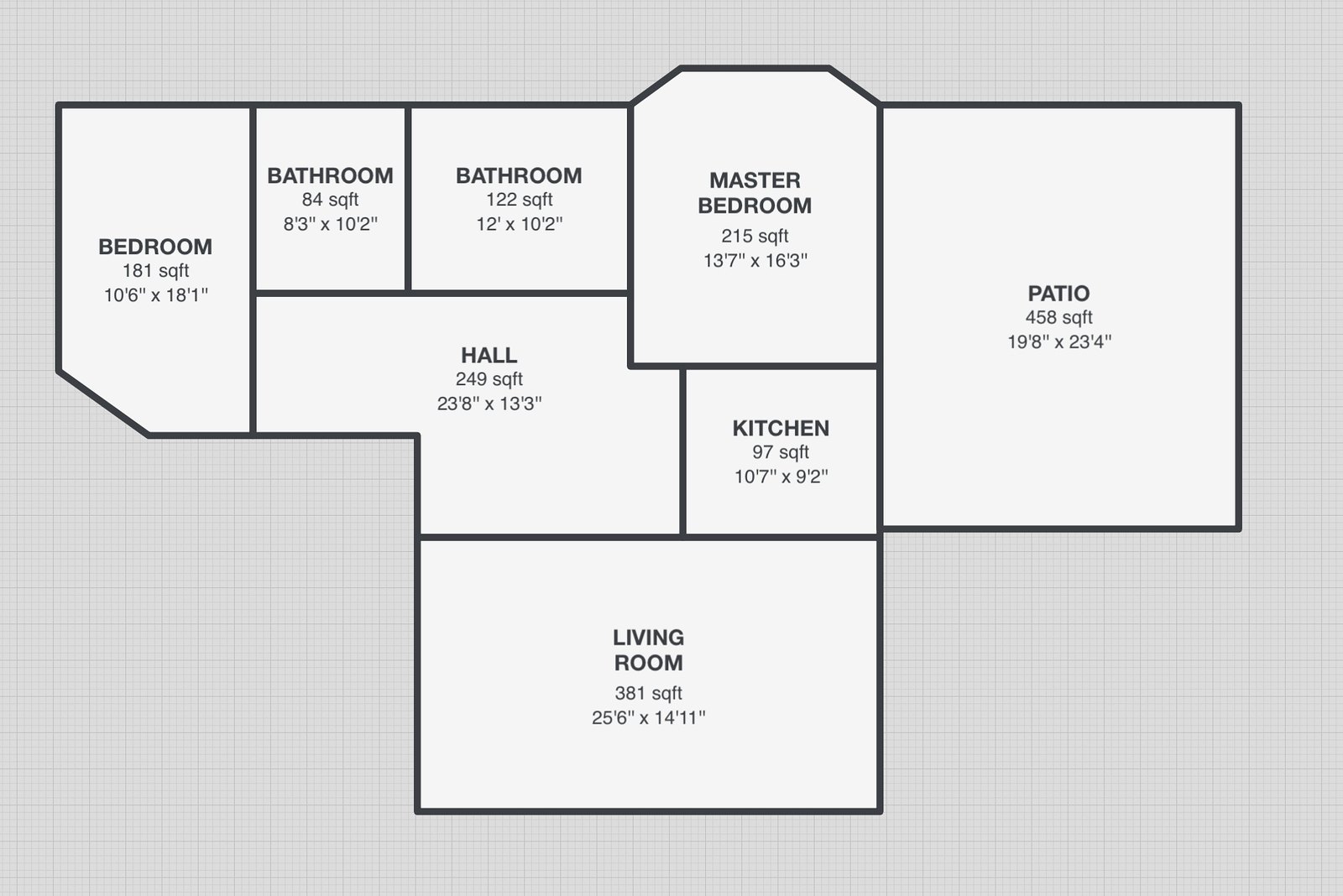This detailed computer-drawn layout depicts the floor plan of a house, set against a gray graph paper background adorned with small squares. The house's structure is outlined in black, with black lettering indicating each room's name, area in square feet, and precise dimensions.

On the far left, a bedroom spans 181 square feet, measuring 10 feet 6 inches by 18 feet 1 inch. Adjacent to this bedroom, moving rightward, is an 84-square-foot bathroom, followed by another bathroom occupying 122 square feet. Below these two bathrooms and to the right of the initial bedroom lies a hallway that covers 249 square feet. 

Notably, the diagram does not indicate any doors or windows, focusing solely on the room layouts which are depicted as squares and rectangles.

Centered at the top of the layout is the master bedroom of 215 square feet. Beneath the master bedroom is the 97-square-foot kitchen. To the right of both the master bedroom and the kitchen is an expansive patio, measuring 458 square feet. Situated at the very bottom of the layout, the living room occupies 381 square feet.

The overall configuration of the house forms a T-shape. The master bedroom notably features a protruding hexagonal area, reminiscent of a bay window's shape, although the diagram does not specify this as a window. Each room's dimensions are meticulously marked with both feet and inches, facilitating a comprehensive understanding of the spatial layout.